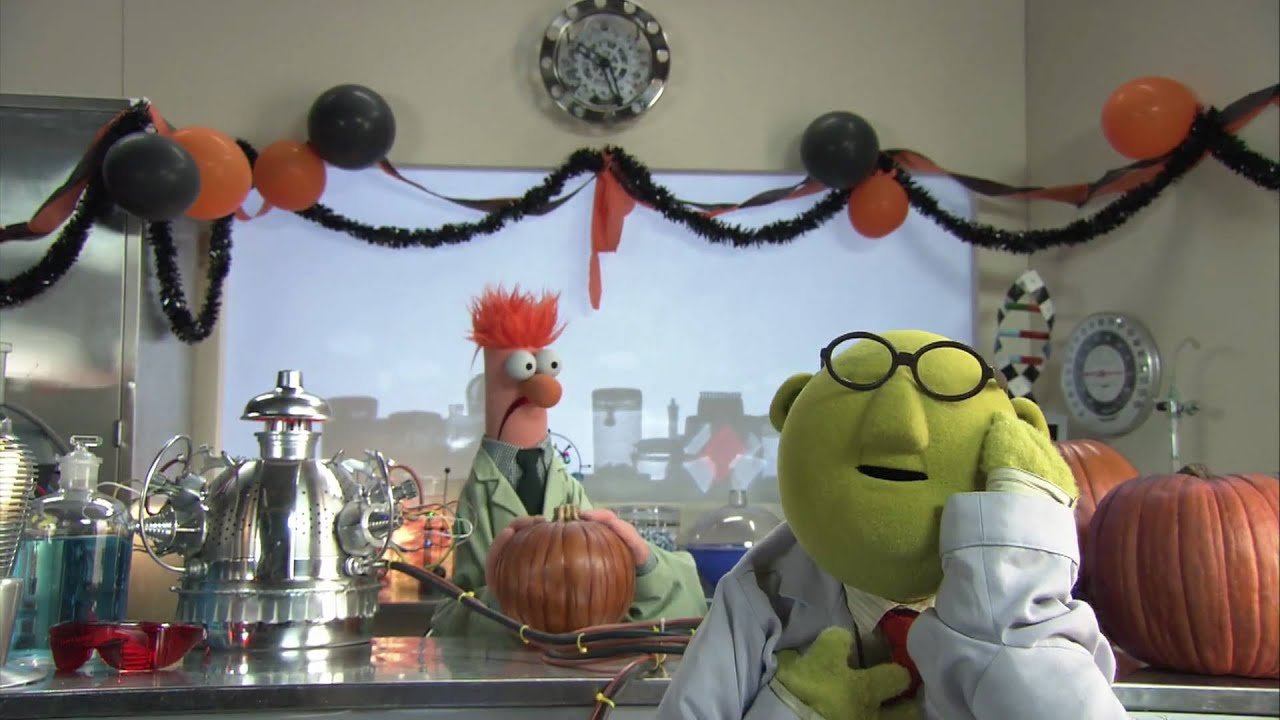This image features a vibrant scene from The Muppets set in a science lab decorated for Halloween. In the foreground, there is a green Muppet with a round head, no visible eyes, sporting black glasses, and wearing a grey lab coat with a white undershirt and a red tie. His hand rests thoughtfully on his face. Behind him stands another Muppet, defined by his cylindrical, narrow pinkish face, spiky bright orange hair, bulging white eyes, and a prominent round pink nose. He wears an olive green lab coat over a grey undershirt and black tie. The lab itself is bustling with Halloween spirit, showcasing numerous pumpkins on the stainless steel countertop, along with scientific equipment like beakers and metal devices. Black streamers, orange and black balloons, and festive decorations adorn the walls, enhancing the lively atmosphere. A double helix model and a steel refrigerator-like appliance are also visible, adding to the scientific setting.